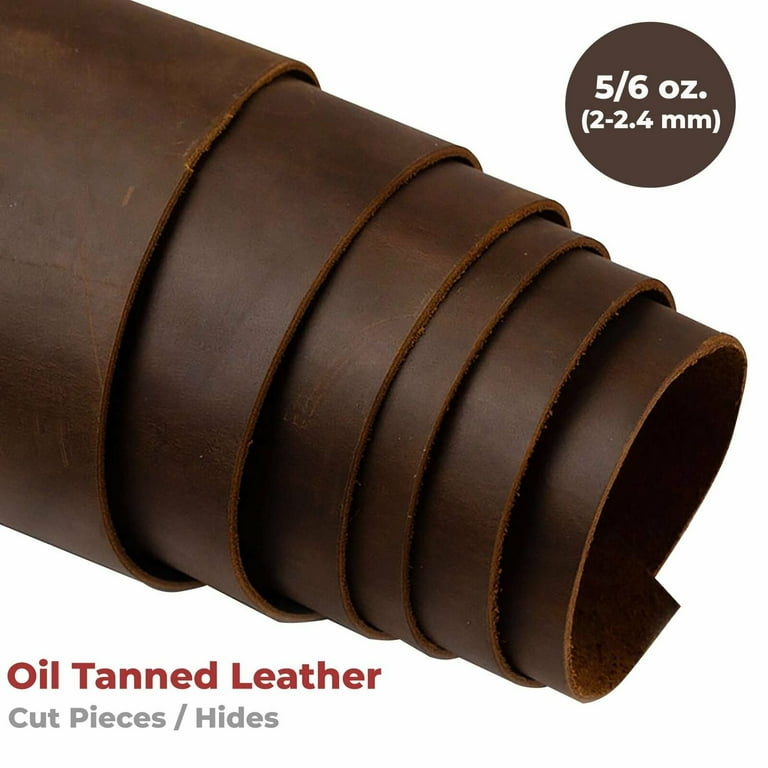The image features a professionally photographed, vertical-rectangular piece of dark brown, oil-tanned leather coiled multiple times, creating a nested appearance against a white background. The composition includes brown text in the bottom left corner stating "Oil Tanned Leather," with smaller gray lettering underneath indicating "Cut Pieces / Hides." In the upper right corner, enclosed in a brown circle, white text specifies "5-6 oz, 2-2.4 mm." The dark brown leather appears shiny, suggesting it has been oiled, and its rich chocolate color varies slightly in the coils. The image seems intended for a website offering oil-tanned leather for purchase, though it does not include company information or a URL.